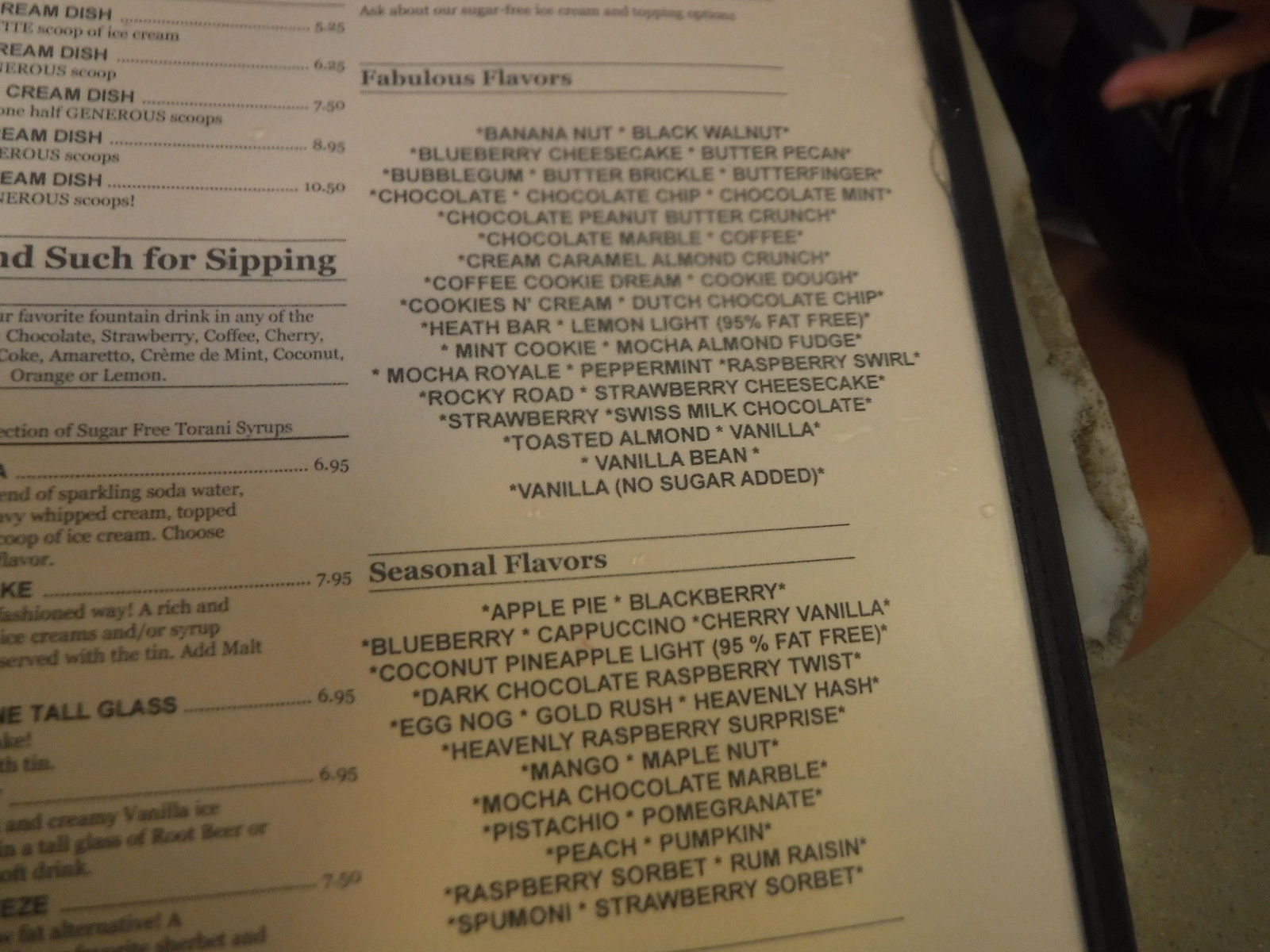The photograph is a rectangular-shaped image capturing a focused section of a menu, specifically highlighting a list of flavors for certain drinks or treats. The menu, primarily out of frame, is a white piece of paper adorned with multiple lines of black text, encased in a holder with black leather-like edges and a clear plastic window. The text on the menu, starting from the right column, lists an array of flavors under the banner "Fabulous Flavors." The flavors include:

- Banana Nut
- Black Walnut
- Blueberry
- Cheesecake
- Butter Pecan
- Bubblegum
- Butter Brickle
- Butter Finger
- Chocolate
- Chocolate Chip
- Chocolate Mint
- Chocolate Peanut Butter Crunch
- Chocolate Marble
- Coffee
- Cream Caramel Almond Crunch
- Coffee Cookie Dream
- Cookie Dough
- Cookies and Cream
- Dutch Chocolate Chip
- Heath Bar
- Lemon Light 95% Fat Free
- Mint Cookie
- Mocha Almond Fudge
- Mocha Royale

The list continues beyond the captured frame, suggesting an extensive selection for patrons to choose from. The photograph emphasizes the rich variety and detail of the offerings.